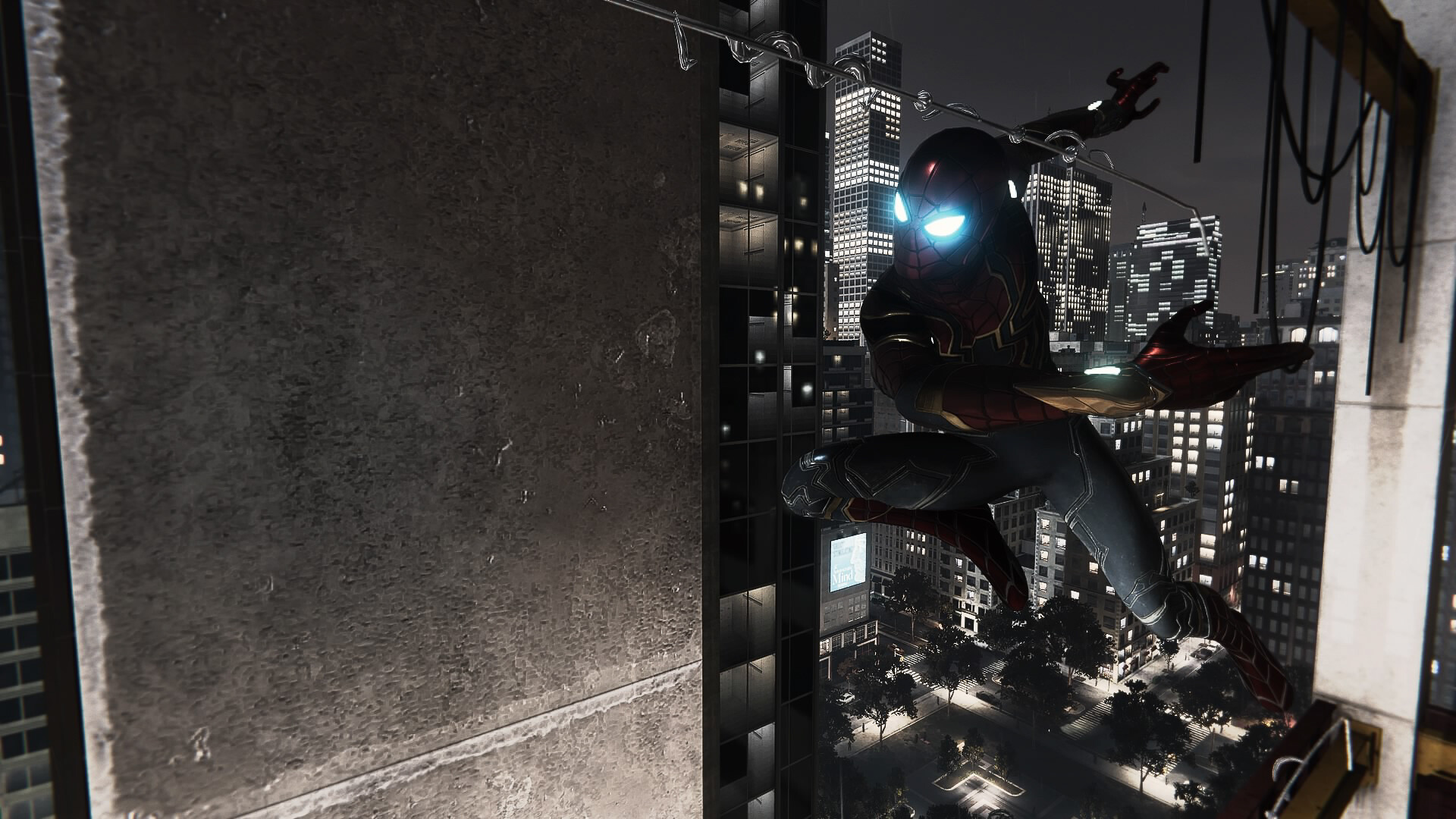In this digitally enhanced, rectangular image set at night, Spider-Man is prominently featured against a backdrop of a cityscape filled with towering, lit-up buildings. The scene suggests a moment from a movie or video game, highlighting Spider-Man in a predominantly dark outfit deviating from his typical bright red, accented instead with deep, shadowy hues. Spider-Man's striking almond-shaped eyes, glowing bright yellow, illuminate his masked face as he appears to be traversing the urban jungle, possibly mid-flight or web-swinging. He clings to the side of a gray concrete building with his hand poised, suggesting impending web action or navigating the space. The detailed scene captures the high-rise buildings and even lower ground elements like trees and landscape lighting, blending realism with the fantastical elements of Spider-Man's world.